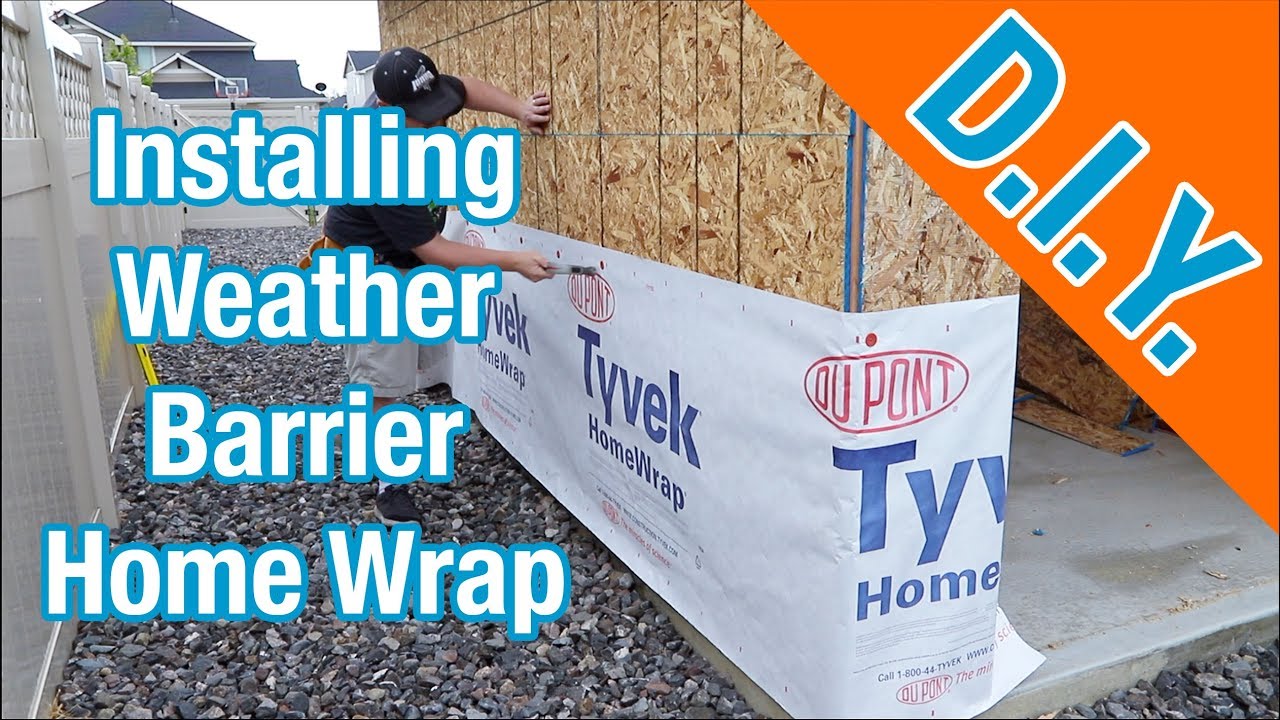This advertisement photograph depicts a construction worker installing Tyvek home wrap, highlighting its use as a weather and vapor barrier for home exteriors. Prominently featured in the upper right corner, an orange triangle with "DIY" in large blue and white block letters emphasizes that this is a do-it-yourself project. Running vertically along the left side, bold white text with blue outlines reads "installing weather barrier home wrap." The scene shows a man clad in a black hat with an embroidered logo, using a hammer in his right hand to secure the Tyvek home wrap onto the unfinished wooden wall of a house. The wrap, branded with "Tyvek" in dark blue letters and "DuPont" in red, contrasts against the white background of the wrap and the light blue measurement lines on the particle board. The setting includes a gravel ground, with a fence featuring a lattice top to the left and other completed homes visible in the background. Tools and lumber scattered around indicate ongoing construction work.